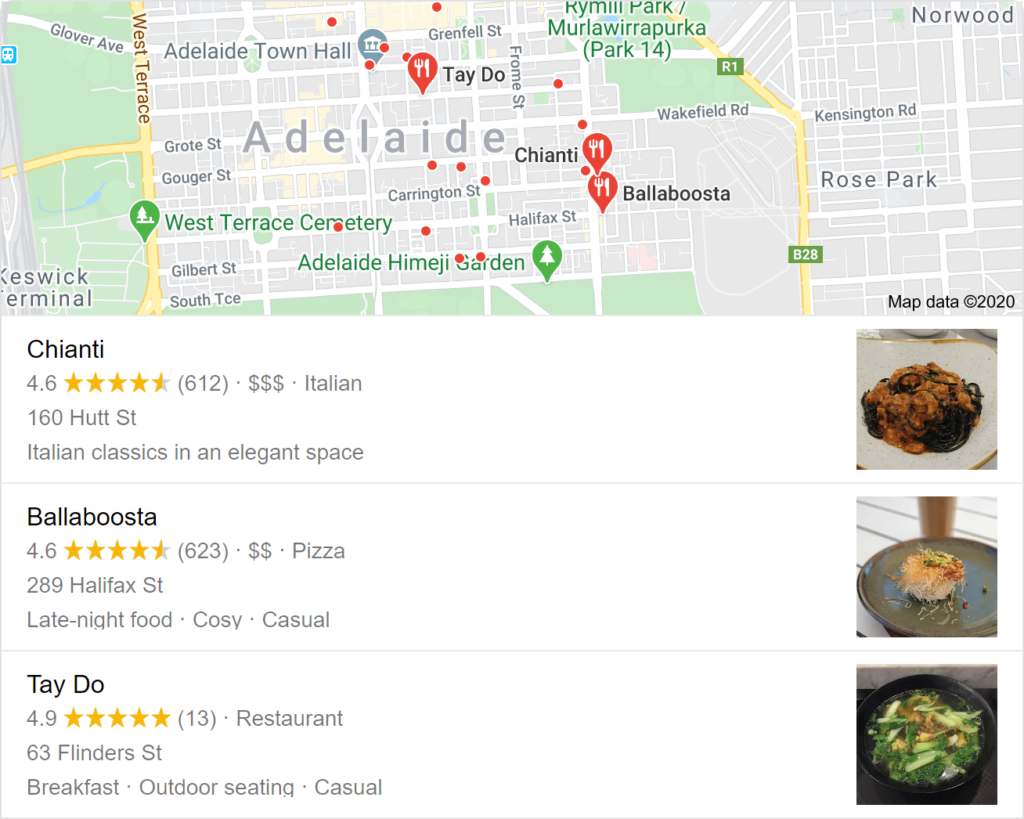This image is a detailed screenshot from Google Maps highlighting dining options in Adelaide, Australia. The map section is dotted with numerous red location bubbles representing various restaurants across the city.

Beneath the map, a list of three prominent restaurants is displayed. The first restaurant, Chianti, is renowned for its Italian cuisine, boasting a high rating of 4.6 stars based on 612 reviews. It is categorized with three dollar signs, indicating a higher price range. The listing includes a visual appeal with a picture of one of their dishes on the far right.

The second listing is Bella Busta, celebrated for its pizzas and rated 4.6 stars from 623 reviews. This restaurant falls into the moderate price range with two dollar signs and is located at 289 Halifax Street. It is noted for offering late-night food and having a cozy, casual atmosphere. An image of one of their dishes, presumably a crab cake on a black plate, is also featured.

The third restaurant, Tay Do, specializes in breakfast options and offers outdoor seating in a casual setting. This establishment has an outstanding rating of 4.9 stars from 13 reviews. Located at 63 Flinders Street, Tay Do’s listing includes a photograph of a dish showing a soup with noodles and spinach.

Each restaurant's entry provides essential information including their star ratings, the number of ratings, price range, type of cuisine, address, and a tantalizing image of a featured dish.